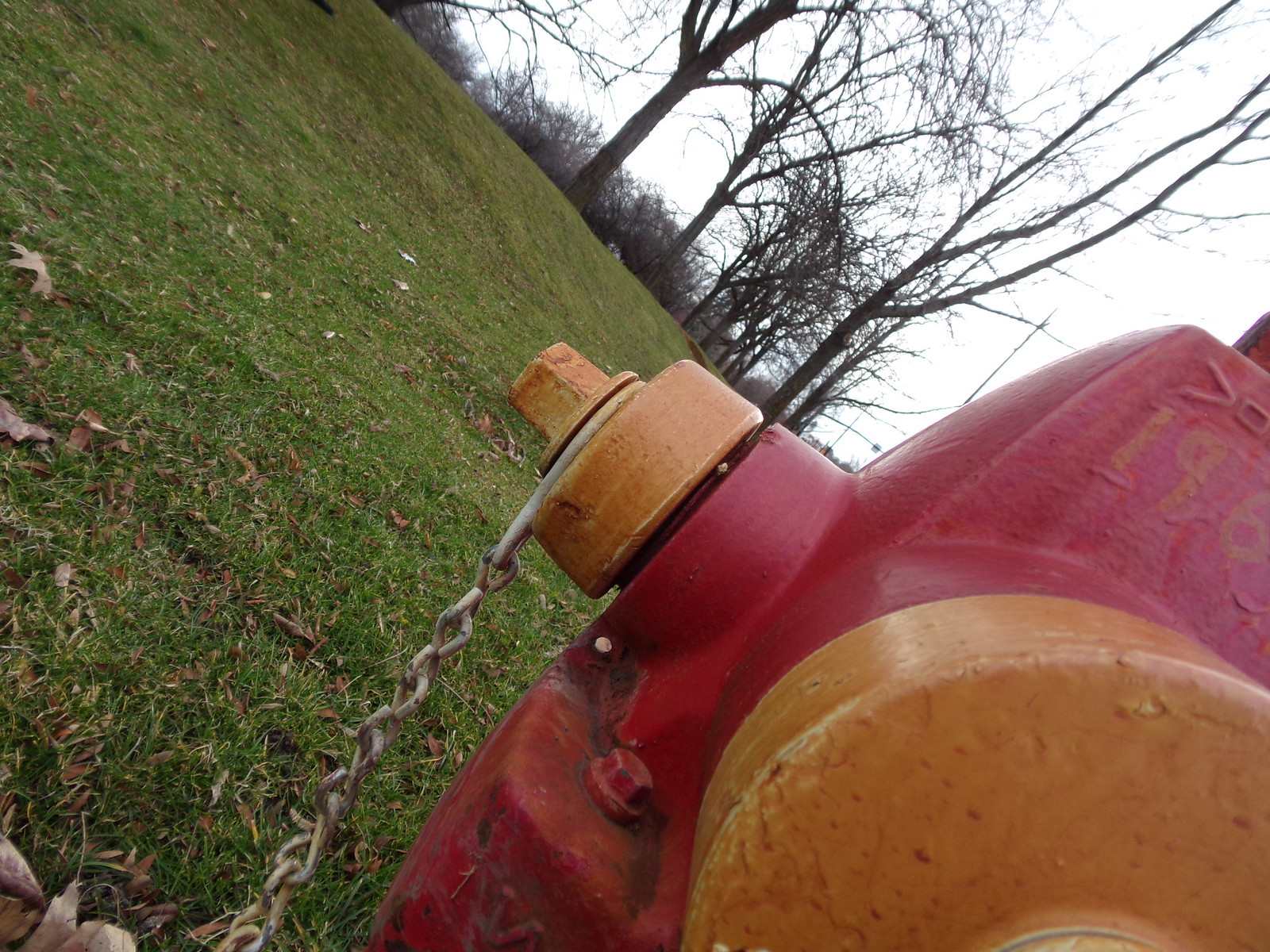The photograph captures an expansive green field with over a dozen leafless trees standing tall in the background, indicating an autumn setting. A pale blue and white sky looms over the scene, giving a light, almost overcast appearance. In the foreground, a slightly dirty, orange and red fire hydrant is prominently featured. The hydrant's red body contrasts with large orange components—a wheel and a valve—where a long chain, tied around one of the caps, dangles down to the ground. The chain lies partially on the grass, which is sprinkled with a few dried autumn leaves. The fire hydrant bears the number "196," partially cropped out of the frame. Small red speckled dots adorn the orange section, adding details to the well-worn fixture. The image's strange angle gives a unique perspective, enhancing the detailed view of the fire hydrant against the tranquil, empty field and barren trees.